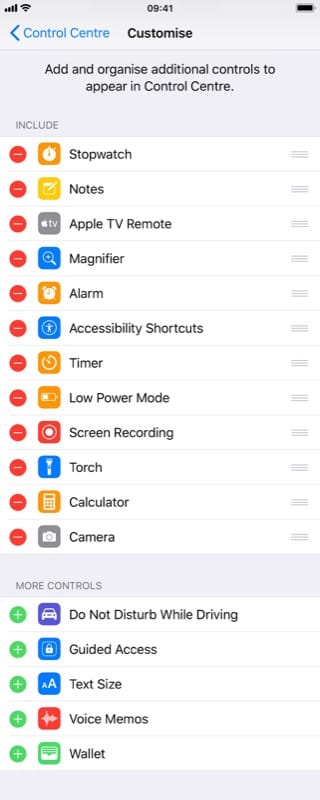This screenshot captures a mobile phone interface depicting a website in portrait mode. The status bar at the top showcases standard icons: Wi-Fi and signal strength on the left, the time (08:40) in the center, and a full battery icon on the right, all in black.

Beneath the status bar is a grey header with "Control Centre" written in blue on the left, accompanied by a back arrow. Centrally placed within the header is the text "Customise," indicating an option to further personalise the Control Centre layout. Below this header, there's an instruction in black: "Add and organise additional controls to appear in Control Centre."

A comprehensive list of apps and functionalities is visible, complete with their corresponding icons and red minus circles to the left of each, suggesting they can be removed from the Control Centre. This list includes:

- Stopwatch
- Notes
- Apple TV Remote
- Magnifier
- Alarm
- Accessibility Shortcuts
- Timer
- Low Power Mode
- Screen Recording
- Torch
- Calculator
- Camera

Following this list, another grey rectangle separates the above sections with the label "MORE CONTROLS" written on it. Below this, additional apps and functionalities are presented with green plus buttons to the left, implying they can be added to the Control Centre. These include:

- Do Not Disturb While Driving
- Guided Access
- Text Size
- Voice Memos
- Wallet

Finally, there is a light grey rectangle at the very bottom of the screenshot, possibly signifying the end of the list or section. The distinction between the red minus symbols and green plus symbols suggests that the former indicates apps currently included in the Control Centre, which can be removed, while the latter indicates apps that are not included but can be added.

Overall, the image clearly represents the customization options available in the Control Centre of an Apple device, even though the observer is unfamiliar with the product interface.